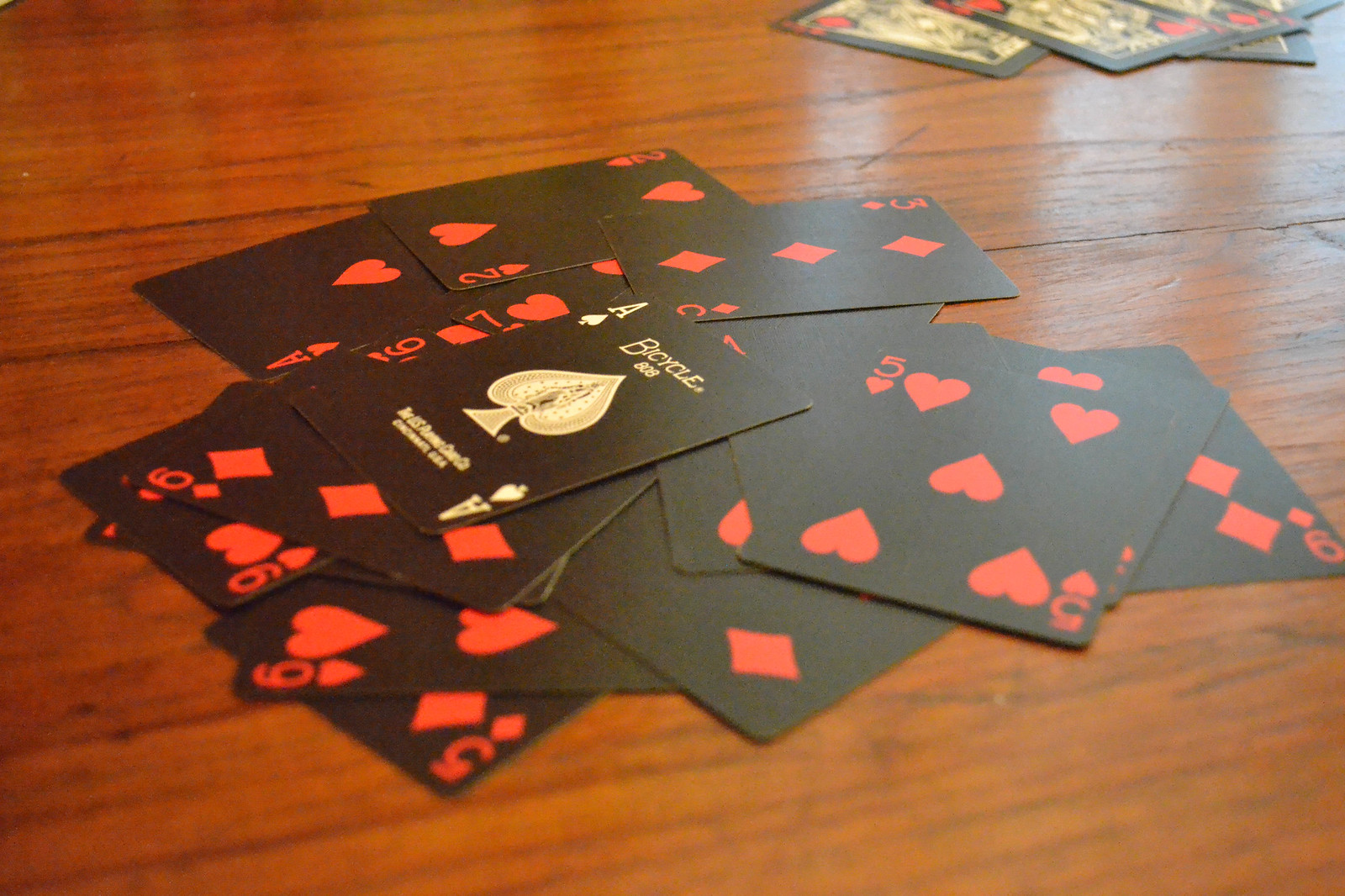A rustic brown wooden table, accentuated with dark grains, serves as the stage for a gathering of playing cards. At the heart of the table lies a deck of predominantly black playing cards, with one card prominently displayed to reveal its back. This card features a sleek black background with the word "BICYCLE" emblazoned in white letters at the top, and a striking white spade symbol centered beneath the text. Each corner of the card showcases a small white ace and spade icon.

Among the scattered cards, the five of hearts is prominently displayed. This card maintains the deck's black background while displaying five vivid red hearts across its face, along with a red numeral '5' and a heart symbol in each corner.

Other cards are strewn to the side, their designs partially visible. These cards share the black rims, yet their centers are white, adorned with various symbols. One visible card is the three of diamonds, featuring three bright red diamonds, with a red numeral '3' and diamond symbol in the corners. Though some cards' identities remain obscured, the splashes of red and white against the vivid black make for a visually striking composition on the wooden surface.